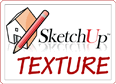The image is a chaotic collage featuring the names of major cities around the world in various white fonts against a sepia-toned background. The city names included are Rome, London, Sydney, New York, Madrid, Berlin, Paris, and Moscow, each occupying distinct rectangular sections within the collage. These names are in different font styles; for instance, Rome and Madrid share a common font, as do New York and Berlin, while London and Moscow have unique fonts.

Each section of the collage includes blurred, off-white images of cityscapes and street signs specific to the named cities, creating an indistinct and chaotic visual effect. Buildings and vehicles are faintly visible in the background, with notable mentions of one-way street signs and multistory buildings with arches in Madrid and Paris. The images blend together, and no individual people stand out. The overall sepia and brown tones lend a modern art feel to the piece, emphasizing the dynamic and bustling essence of urban environments around the world.